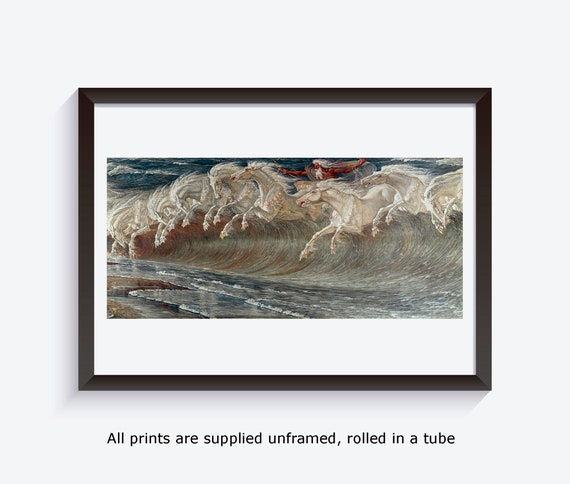This product advertisement showcases a famous painting by Walter Crane called "Neptune's Horses." The artwork is displayed in a simple black frame and depicts an imaginative oceanic scene where the crests of stormy waves transform into a procession of white horses, surging towards a beach under a blue sky. Hovering majestically above these waves is Neptune, the sea god, distinguished by his long white hair and beard, with his dark red skin contrasting against the dynamic scene. The powerful imagery of the white horses merging with the waves features striking blue and reddish streaks throughout the water. Below the painting, there is informational text indicating, "All prints are supplied unframed, rolled in a tube."